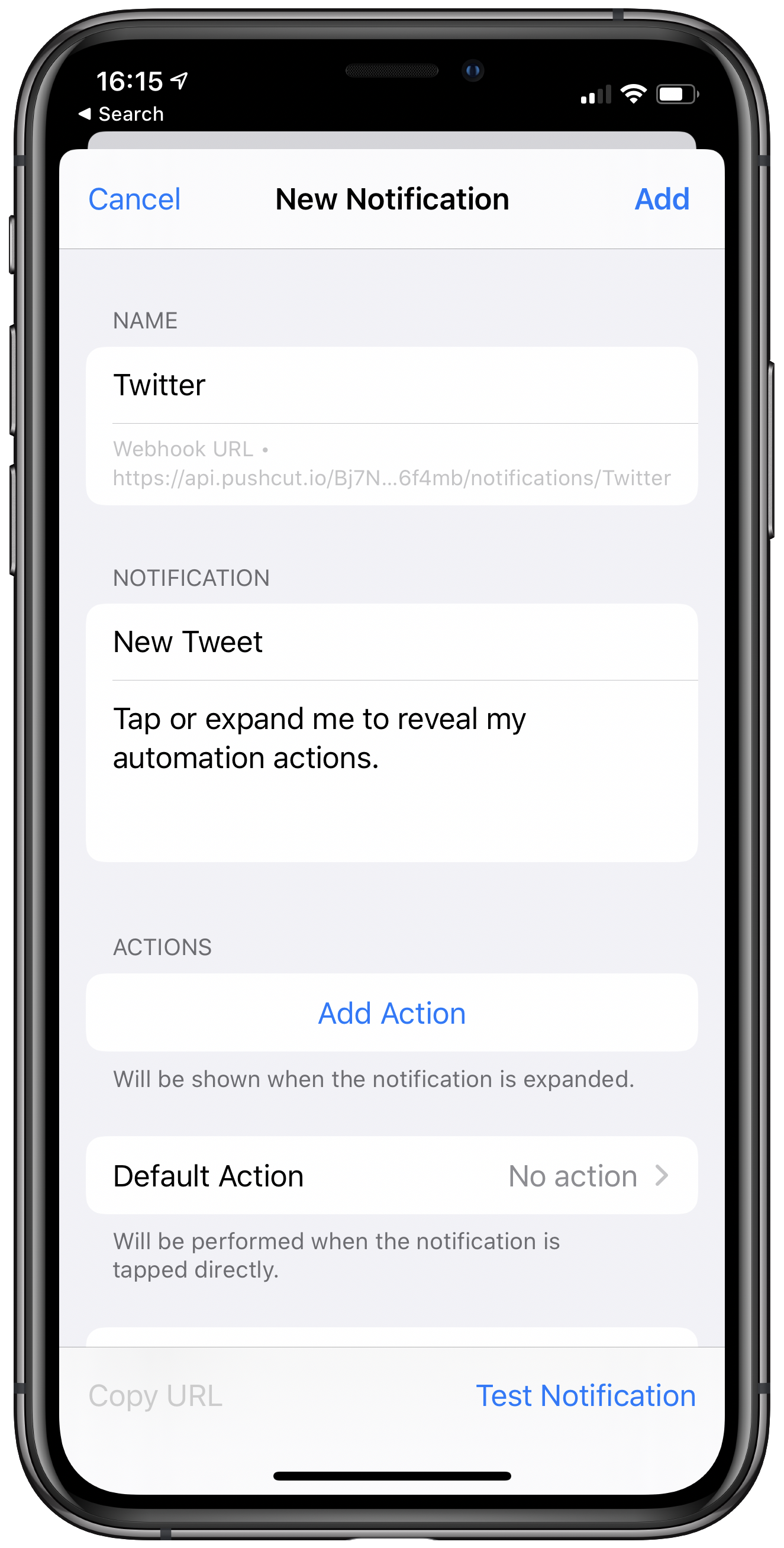In this image, we see a black cell phone with its screen turned on, displaying a detailed interface. The phone is positioned upright, with its height being greater than its width. The screen features a black background with white text indicating the time as 16:15. Beneath the time, there's an arrow pointing left accompanied by the word "Search." 

In the top right corner of the screen, status icons indicate the phone's connectivity and power status: two bars signify network signal strength, a lit Wi-Fi icon confirms connection to a Wi-Fi network, and a battery icon shows the remaining battery life.

The physical features of the phone include three buttons on the left side. The top button is noticeably the smallest, while the two buttons below it are of equal length. On the right side of the phone is a single, long button.

On the screen, a notification panel creates a contrast with its white background. The top line reads "New Notification," accompanied by a blue "Cancel" button on the left and a blue "Add" button on the right. The notification lists "Name: Twitter" and "Notification: New Tweet." The message invites the user to "Tap or expand me to reveal my automation actions." 

Towards the lower part of the screen, there is a button labeled "Add Action." On the bottom right of the screen is another button labeled "Test Notification" in blue text, ready to be interacted with.